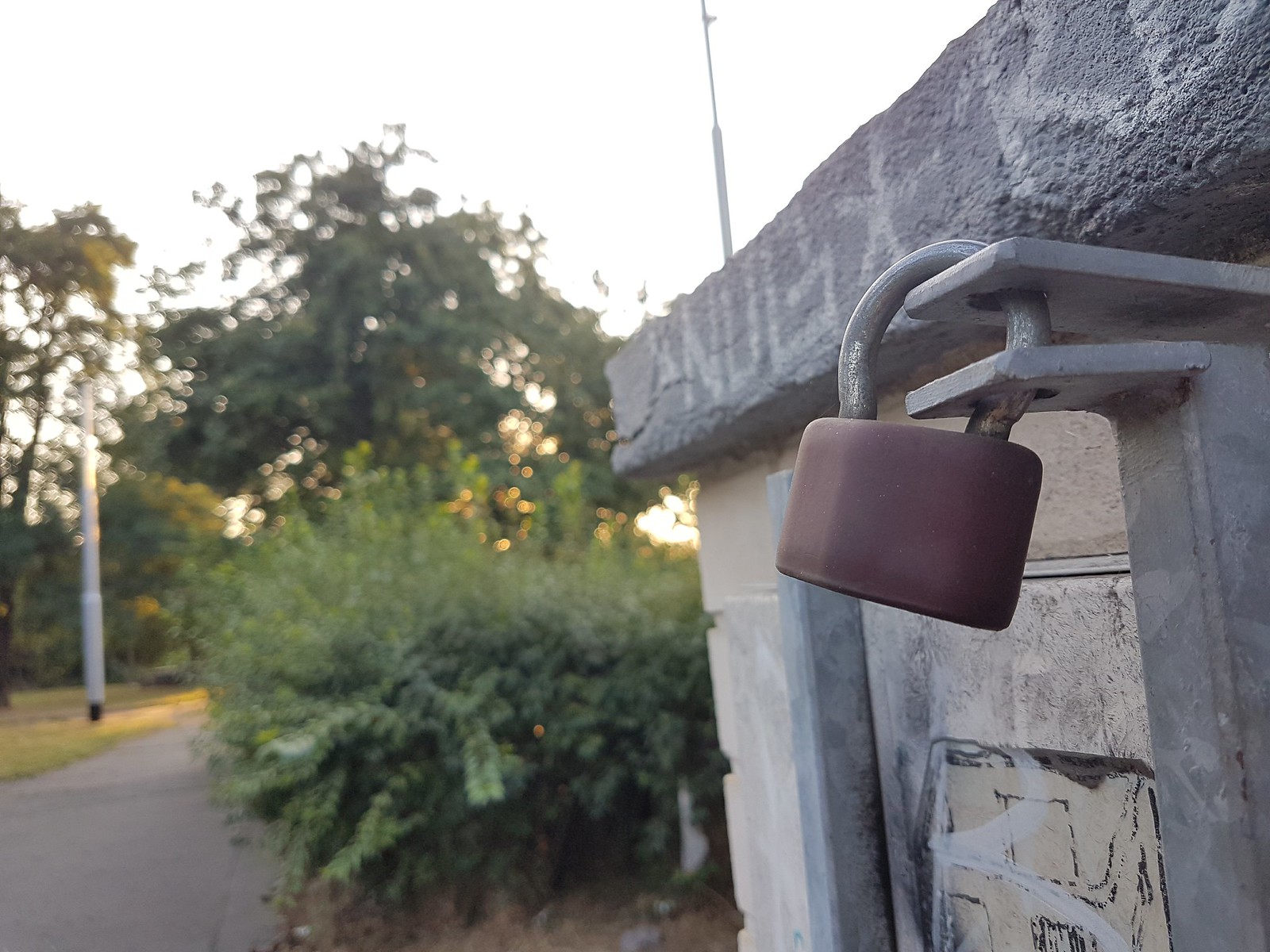The daytime outdoor photograph captures a concrete walkway flanked by green shrubs and trees, indicative of a park or nature trail setting. Situated next to the walkway is a small concrete structure with a metal barred door. The bars, made of square metal tubing, are secured at the top with a red plastic-covered lock, ensuring weather protection. The lock connects through a flange with holes that align the bars. The structure features some graffiti on its concrete roof and a strip of white, undecipherable text suggesting weathering or an unmaintained state. The predominant hues in the image include shades of green from the foliage, various greys from the concrete and stone, and reddish tones from the lock. Overall, the scene suggests a serene but somewhat neglected public space, with the setting being during daylight, potentially morning or late afternoon.